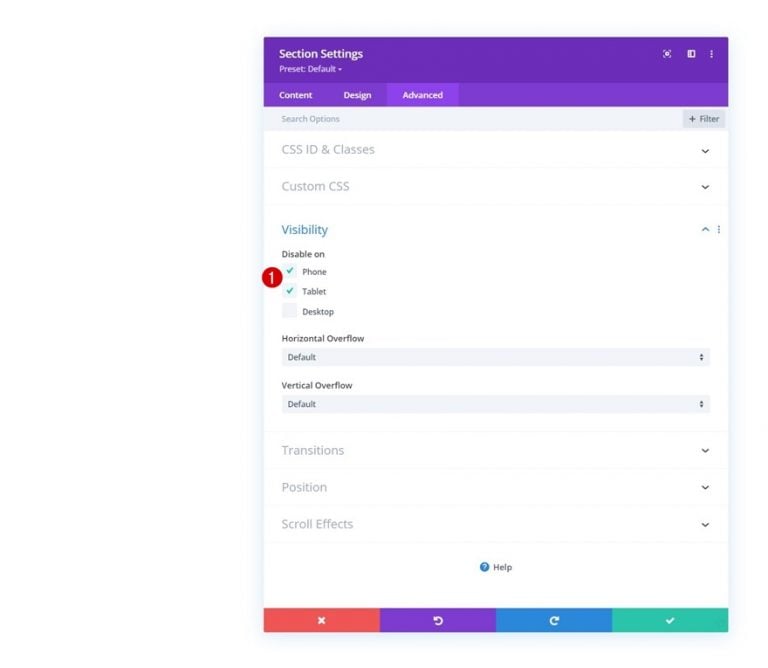The image displays a website design application's 'Section Settings' interface. The screen is divided into two sections: the upper portion has a blue and purple gradient background, while the lower section is white. At the top of the interface, the label 'Section Settings' is clearly visible. Below this, there are four main tabs: 'Default', 'Content,' 'Design,' and 'Advanced', with 'Advanced' currently highlighted and active.

Within the 'Advanced' settings, various configuration options are presented. These include fields for 'CSS ID and Classes', 'Custom CSS', and 'Visibility.' The 'Visibility' option is expanded, revealing checkboxes for 'Disable on Phone', 'Tablet', and 'Desktop'. In this case, visibility is disabled on both phone and tablet. The 'Horizontal Overflow' and 'Vertical Overflow' settings are both set to 'Default'. Other notable options within the 'Advanced' tab include 'Transition', 'Position', and 'Scroll Effect.'

At the bottom center of the interface is a 'Help' icon, represented by a blue question mark. Along the bottom of the screen, there are four functional icons: a red 'Close' icon (an X), a purple 'Undo' icon, a blue 'Redo' icon, and a green 'Accept' icon (a checkmark), positioned from left to right. The detailed interface allows the user to refine and customize the settings and preferences of the website, with the 'Advanced' section prominently displayed in this example.